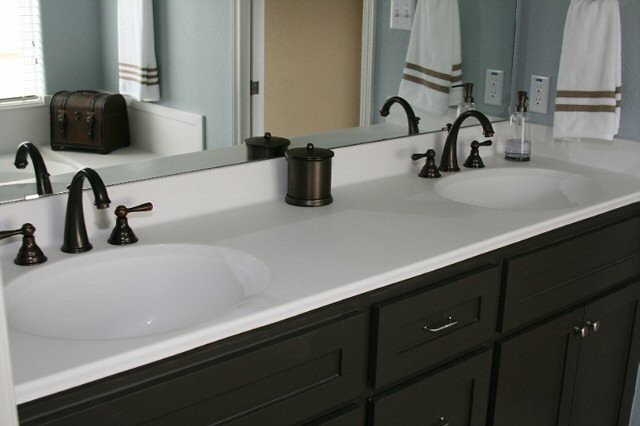This is a detailed color photograph showcasing a bathroom sink and counter area featuring a seamless blend of modern and classic designs. The setup includes a double sink arrangement with a smooth, shiny white countertop neatly separating the two basins. Each sink is equipped with dark bronze faucets and handles that stand out against the pristine white surface. Both sinks are currently turned off.

Positioned centrally, nestled against a large mirror, is a circular container rendered in matching dark bronze, complete with a lid and a small round knob. To the right of the second basin, a clear pump bottle with a bronze-colored top sits partially filled with what appears to be white or clear liquid soap.

The bathroom's walls are painted a calming shade of gray, harmonizing with the minimalist yet elegant decor. In the upper right corner of the image, a white towel accented with two horizontal brown stripes is visible. Below the sinks, dark wooden cabinets with sleek silver handles and knobs offer a rich contrast to the light countertop.

The mirror provides a reflective glance into the room, revealing more of the dove gray walls. Reflected in it, there's a small suitcase, another matching striped towel, and the edge of an open doorway, adding depth and an element of lived-in comfort to the space.